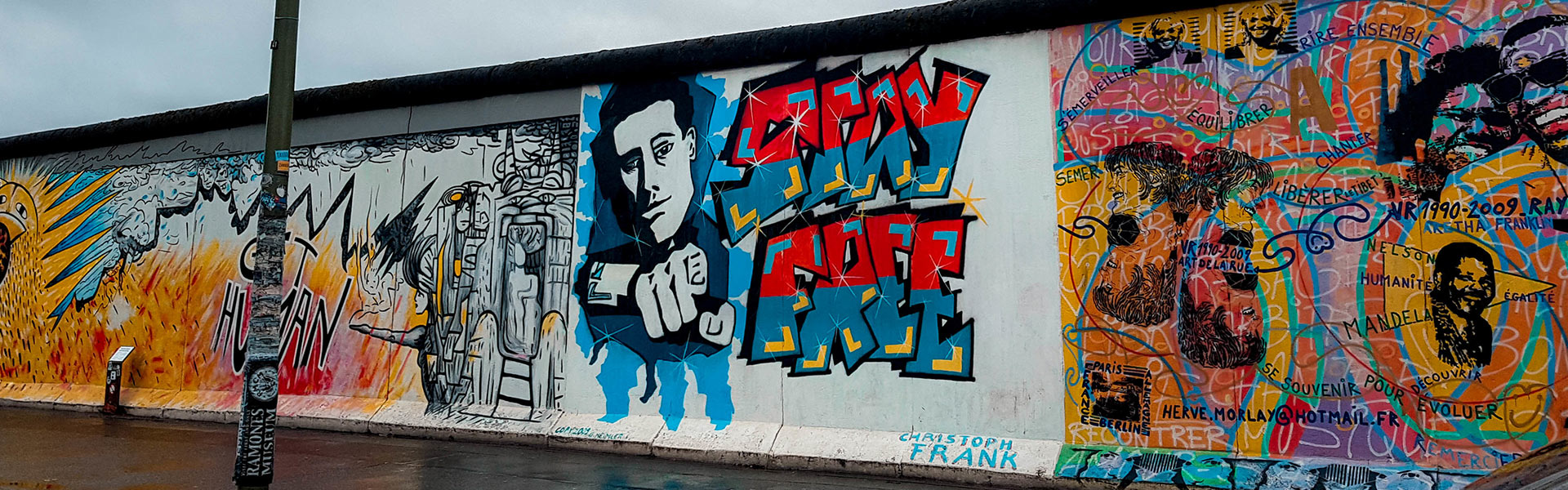This is a horizontally oriented photograph capturing a vibrant city street scene with a long, gray wall adorned with eye-catching graffiti and murals. The outdoor setting is illuminated by a clear blue sky dotted with white clouds. The wall, approximately 10-12 feet high, boasts three distinct pieces of street art created by different artists.

On the left side of the image, a colorful mural featuring abstract shapes and vibrant hues can be seen. Adjacent to this, another mural prominently displays the phrase "Stay Free" in red, blue, and yellow text. This mural includes a striking image of a man pointing directly at the viewer, adding a dynamic and engaging element to the art. The piece is signed by the artist Christoph Frank.

Moving to the right side of the photograph, there's a mural that acts as a tribute to various influential African Americans throughout history, including Ray Charles and Nelson Mandela. This section is particularly colorful, with a mix of blue, red, and orange hues, and vividly painted portraits of numerous famous figures. One piece of text reading "Get Human" is visible amid the patterns that might symbolize fire. An email address is noted at the bottom of this section, although it's partially obscured.

In front of the wall stands a light pole, adorned with assorted stickers, adding another layer of urban character to the scene. The combination of these elements creates a rich tapestry of cultural and artistic expression, vividly portrayed on this expansive outdoor canvas.